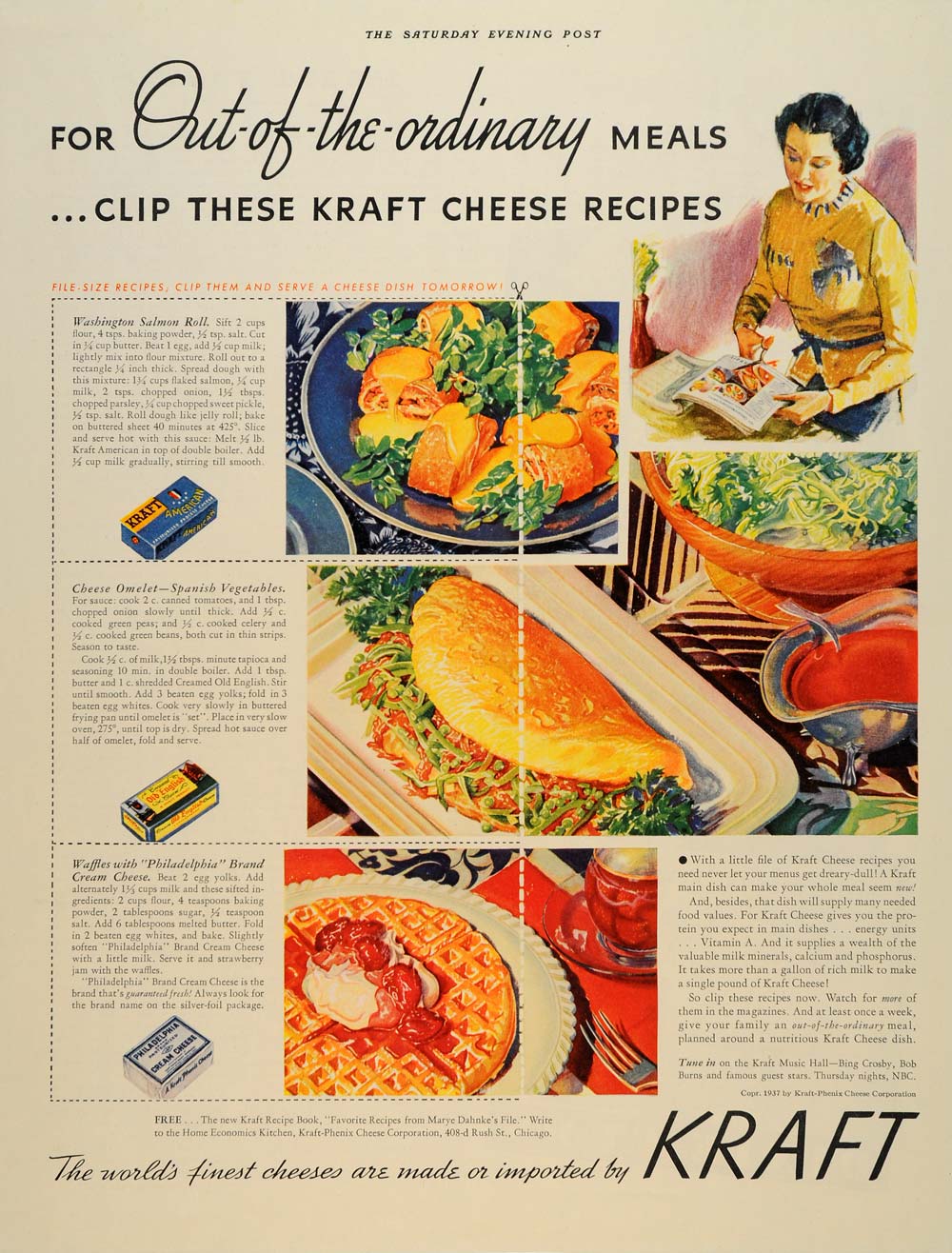This image is a meticulously detailed advertisement page from a 1950s issue of The Saturday Evening Post, promoting Kraft cheese. The page headline, prominently displayed in large, bold font, reads, "For Out of the Ordinary Meals Clip These Kraft Cheese Recipes." Beneath this title, colorful illustrations showcase an array of recipes ingeniously incorporating Kraft cheese. Highlighted dishes include Washington Salmon Roll enveloped in cheese, a hearty cheese omelet with Spanish vegetables, and an innovative waffle served with Philadelphia brand cream cheese. The upper right corner features a 1950s housewife illustration, depicting her clipping a recipe from the magazine. The ad emphasizes the quality of Kraft's cheese, noting that the world's finest are made or imported by Kraft. Overall, this nostalgic advertisement cleverly intertwines practical recipes with appealing visuals, exemplifying Kraft’s mid-century marketing appeal.